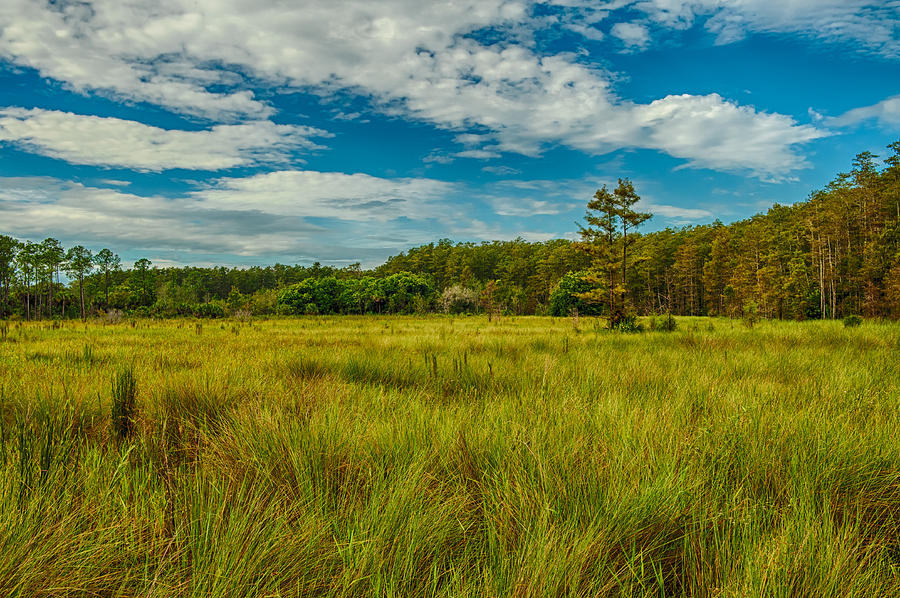This image captures a vibrant and expansive grassy field that stretches into the horizon. The foreground is dominated by tall grass, exhibiting a palette of greens, yellows, and light browns, suggesting a windy day as the blades appear to be swaying. Toward the center right of the image, just slightly to the right of the middle, stands a lone tree, mingling within the sea of grass. The scene transitions into a dense forest spanning the background, showcasing a variety of trees with differing heights and widths—some are tall and slender while others are short and bushy. The forest visually thickens towards the right side of the photo. Above, the sky is a radiant, enhanced shade of blue, adorned with white clouds that drift diagonally from the upper left to the middle of the right side. The enhanced colors of the scene give it a slightly surreal quality, intensifying the natural beauty and contrasting the vivid green and yellow hues of the field with the bright blue and fluffy white of the sky.